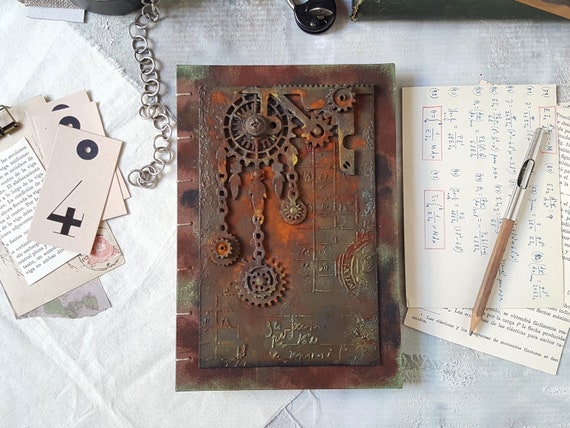The image showcases a steampunk-inspired artwork meticulously assembled on a white cloth surface. At the centerpiece is a brown, metallic rectangular box, reminiscent of an old-school notebook, featuring a rusty texture with bronze hues and a patina of verdigris, suggesting aged metal. The box is adorned with an intricate array of gears, mechanical parts, and embossed embellishments giving it a pronounced 3D effect, intertwined with chains and motors, and covered with an array of engraved writing. 

To the right of the box, several pieces of paper are visible, including one filled with numerous math equations in blue ink interspersed with red squares, partially concealing another sheet with more handwritten notes. A pencil, brown at the tip and silver at the end, rests atop the papers. To the left of the central box, there are small rectangular paper tags with numbers and letters, possibly part of a cataloging or timekeeping system, attached to a silver chain, enhancing the industrial theme. The setting is awash with natural light, adding a simplistic, yet organized feel to the otherwise intricate and detailed composition.